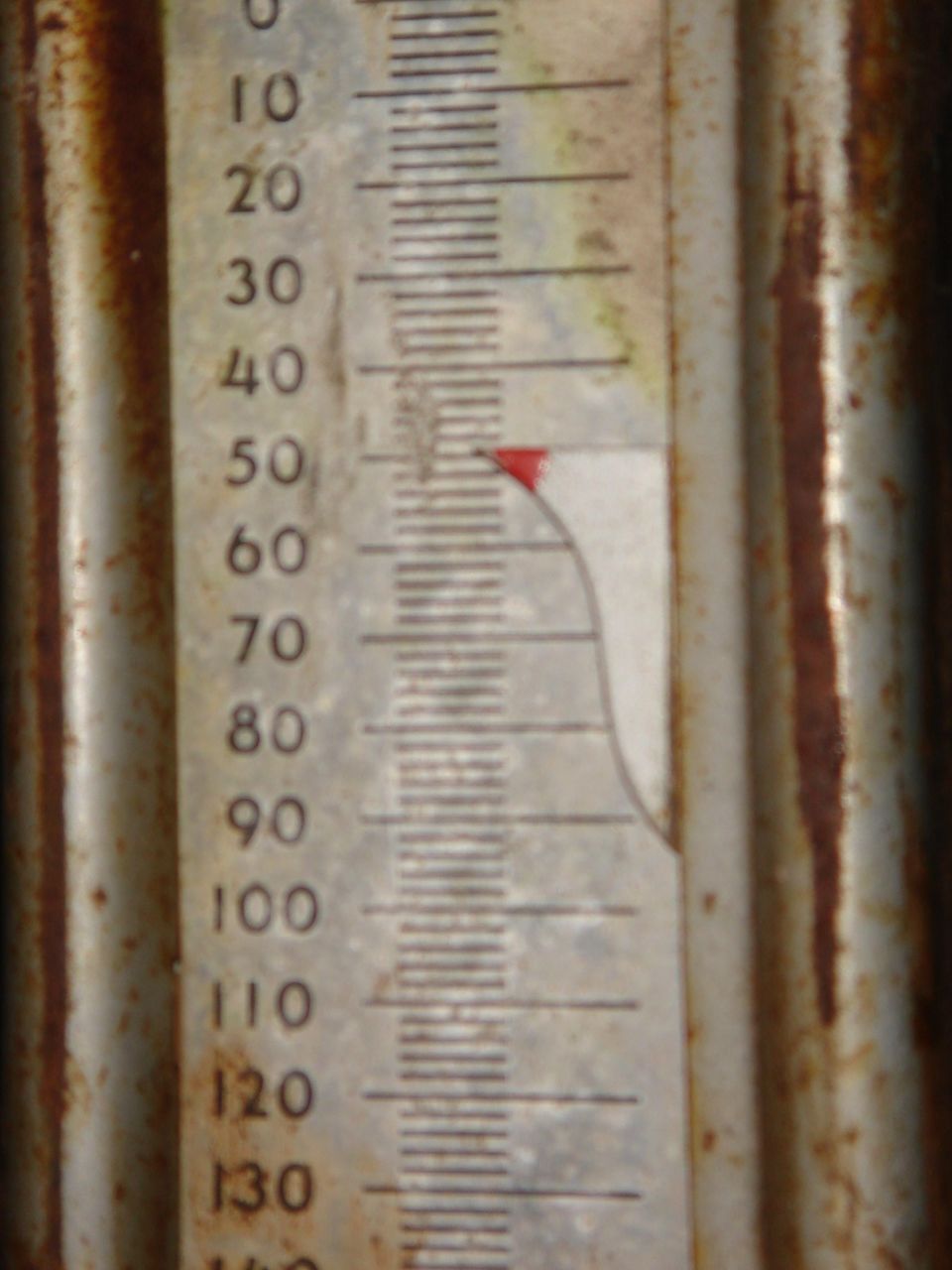In this image, we see what appears to be a highly corroded thermometer. The device is primarily silver, but extensive rusting has occurred, leaving long streaks and small, circular patches of brown rust across its surface. Starting from the top and moving down the center, we observe a series of markings and numbers. On the left, the scale begins at zero, followed by four short lines, each approximately an inch and a half to two inches long. Beneath these lines, the number 10 is marked next to a longer line. This pattern continues with the numbers 20, 30, 40, and 50, each accompanied by a prolonged line and four shorter lines between them. At the 50 mark, a red-tipped white rectangle or square is positioned precisely at the end of this long line, likely indicating the current measurement. The scale proceeds downwards, extending to 130, with a glimpse of what is likely the number 140 at the very bottom. This intricate detailing and the presence of the old, mechanical structure suggest this is possibly an antiquated type of thermometer.